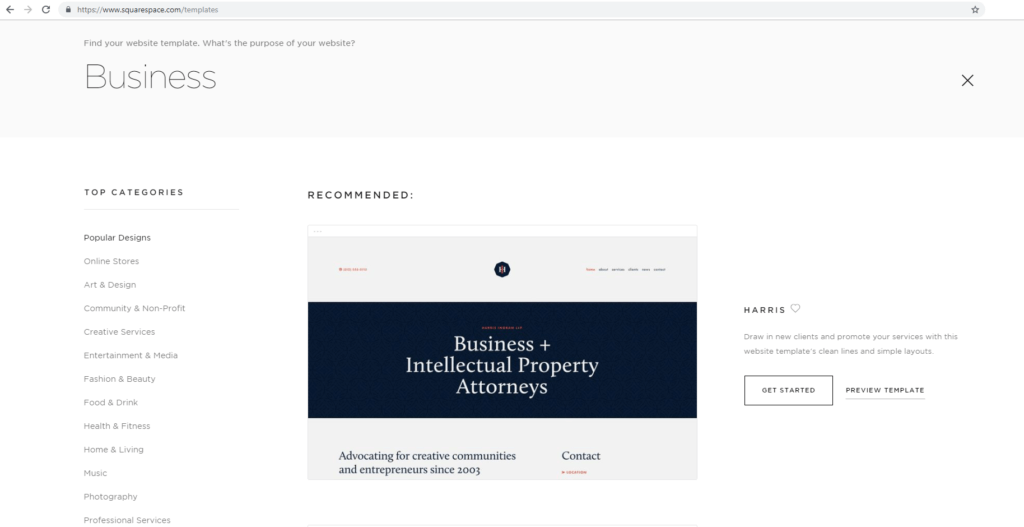A screenshot of the top section of a webpage from Squarespace.com, specifically from the "Templates" section. The URL displayed is "squarespace.com/templates," and the heading at the top of the page reads, "Find Your Website Template." The website's purpose, indicated as business-oriented, is showcased with various design categories on the bottom left-hand side. These categories include Popular Designs, Online Stores, Art and Design, Community and Non-Profit, Creative Services, Entertainment and Media, Fashion and Beauty, Food and Drink, Health and Fitness, Home and Living, Music, Photography, and Professional Services.

The middle section features a "Recommended" label, alongside a box containing a smaller black bar, suggesting a highlighted template for business intellectual property attorneys. On the bottom right-hand side, there's an ad for hair mousse, accompanied by a small heart icon. The webpage encourages users to "Draw in new clients and promote your services with website templates," emphasizing clean lines and simple layouts. Additionally, there are interactive options with a boxed "Get Started" button and an underlined "Preview Template" link, guiding users through the initial setup of a Squarespace business website.